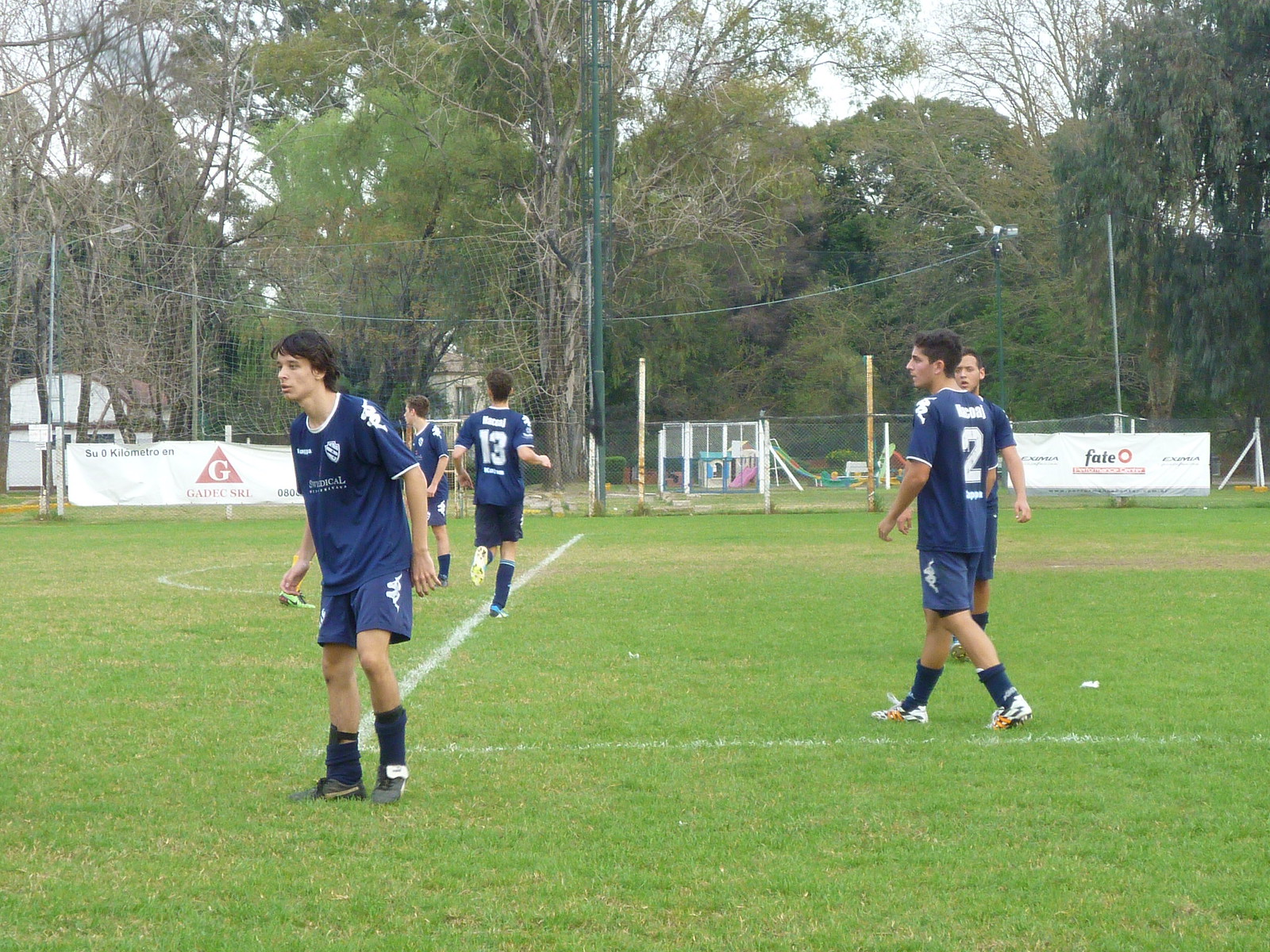The photograph depicts a group of young men in their late teens, clad in dark navy blue soccer uniforms which feature white logos and collars. They are assembled on a well-maintained grassy field marked with white chalk lines, indicative of a soccer practice session. The players are engaged in various activities; one is running while others are walking or standing, suggesting they are at practice rather than in the midst of a game, as no soccer ball or opposing team is visible. The scene is set against a residential backdrop, where a chain-link fence adorned with advertising banners—one showing a triangle with the letter "G" and another partially readable banner stating "fate O"—separates the field from the background. Behind the fence, the area transitions into a residential neighborhood with visible structures such as a small playground featuring a plastic slide and two houses. Tall trees, a mix of lush green and bare-branched, tower in the far background, implying an early spring day. The practice field also includes a distant soccer net, further emphasizing the training setting.